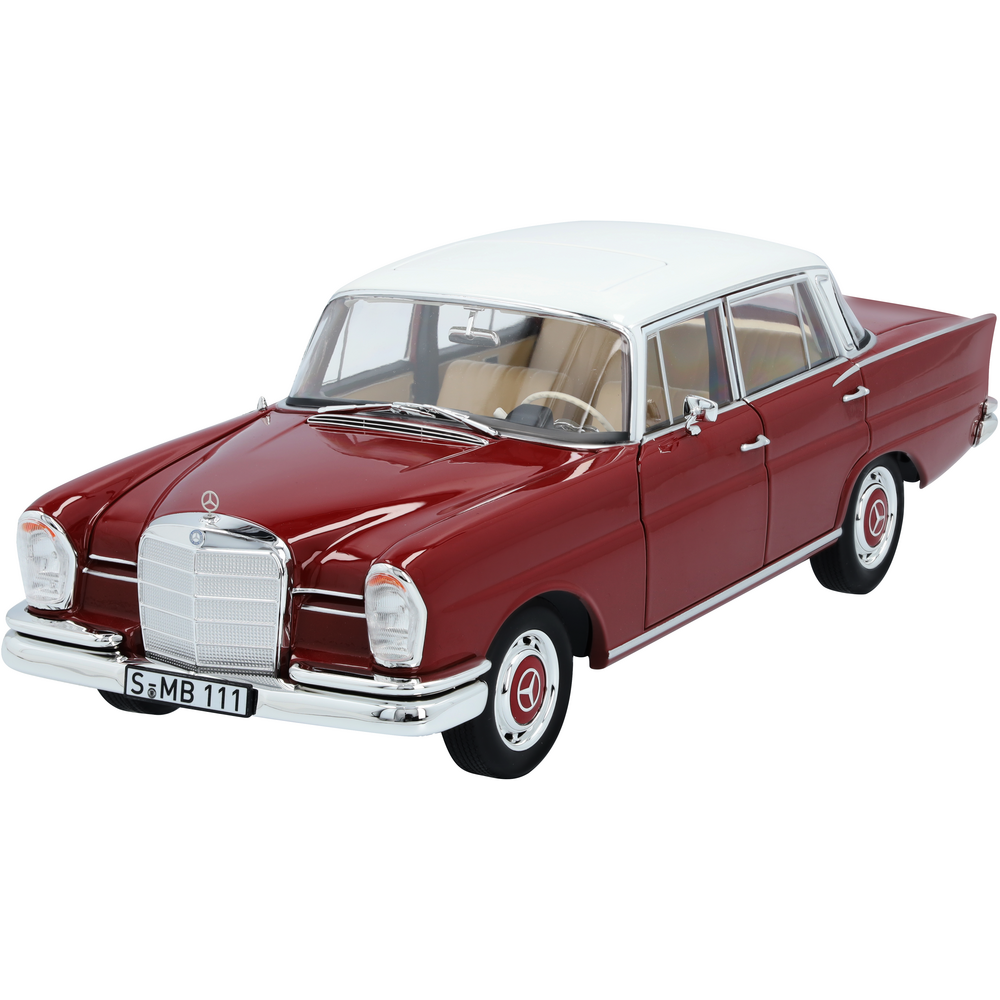In this image, a detailed die-cast model of a classic, cherry-red Mercedes-Benz is showcased with no background, making the car the sole focus of the photograph. The model boasts a white roof and a highly detailed beige leather interior, including a white steering wheel and a silver mirror hanging down from the center console. The front of the car features a distinctive grille in silver and white, accompanied by silver bumpers at both the front and rear. A vintage feel is given by the well-kept black tires, which have silver rims with a red center, sporting the iconic Mercedes-Benz emblem. The license plate displays "S-MB 111" in black text on a white background, indicating a European origin. Further details include white lights and a detailed ornament on the hood, which consists of a circle traversed by three lines, solidifying its classic aesthetic. The exceptional craftsmanship of this toy car makes it appear almost lifelike, hinting at the luxurious design of an actual 1950s era vehicle.